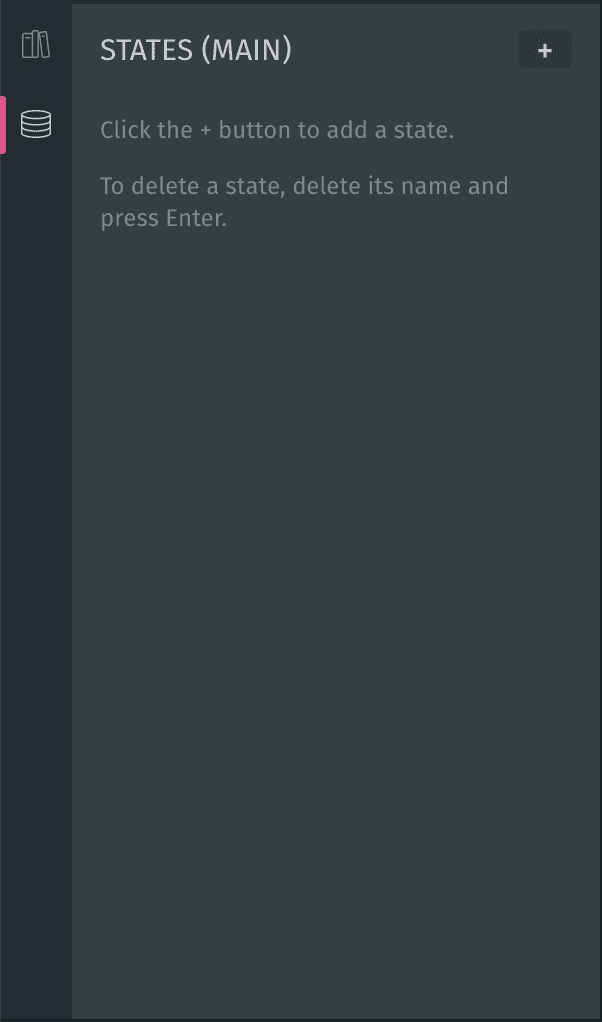The image depicts a webpage with a minimalist and clean interface. The central focus is a section titled "States: Maine." Below this title, there is an instructional text that reads, "Click the plus button to add a state. To delete a state, delete its name and press enter." The background of the page is a neutral gray, providing a subtle and unobtrusive backdrop. There are no additional elements or distractions present on the page, emphasizing the simplicity of the interface.